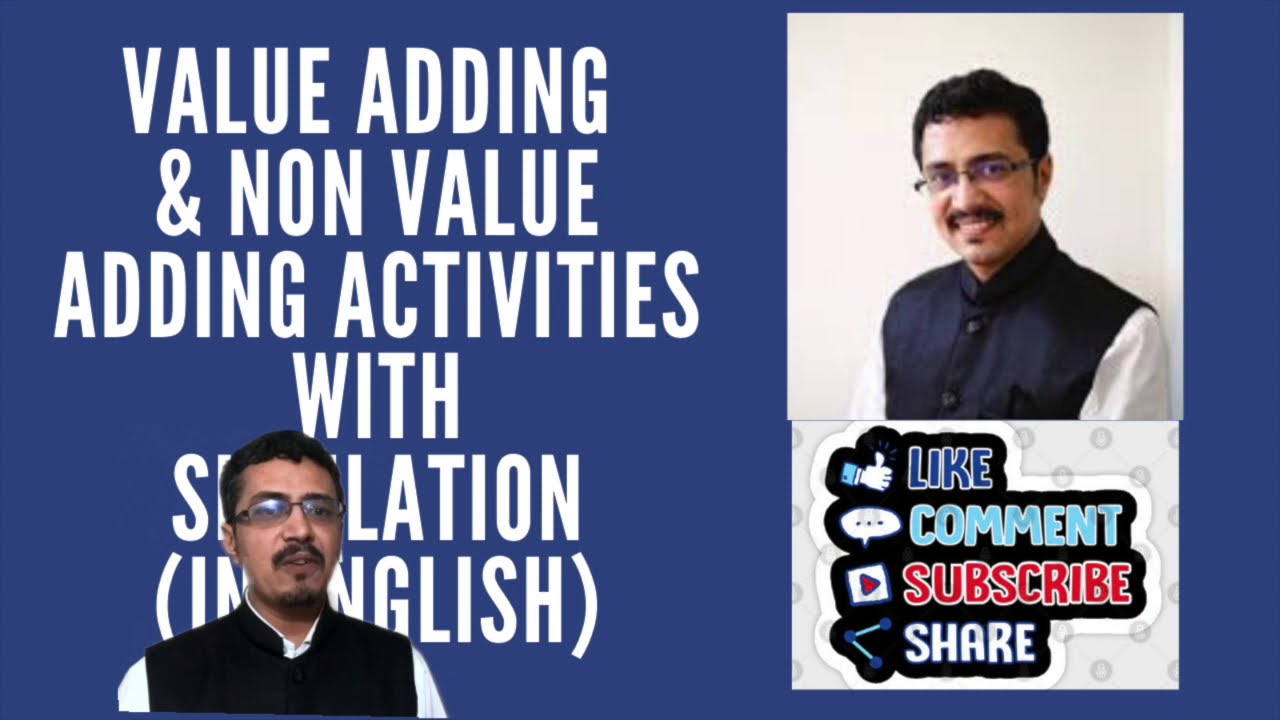This is a wide, rectangular image, possibly a screenshot from a website or YouTube channel, featuring a man of Indian descent with short black hair, glasses, and a mustache. The man, dressed in a white shirt and a dark vest (described variously as black, navy blue, or purple), is positioned in the bottom left corner, visible only from the shoulders up. He is looking directly at the camera. On the left side of the image, a blue background displays text in thick, all-capital white letters that read "VALUE-ADDING AND NON-VALUE-ADDING ACTIVITIES," followed by partially obscured words that end in "LATION." Underneath, in parentheses, appears the fragment "(...GLISH)." The top right corner of the image contains a smaller square photo of the same man, smiling towards the camera. Below this photo, there are colorful, uppercase prompts to "LIKE" (with a thumbs-up icon), "COMMENT" (with a speech bubble icon), "SUBSCRIBE" (with a heart icon), and "SHARE" (with a graph-like icon).